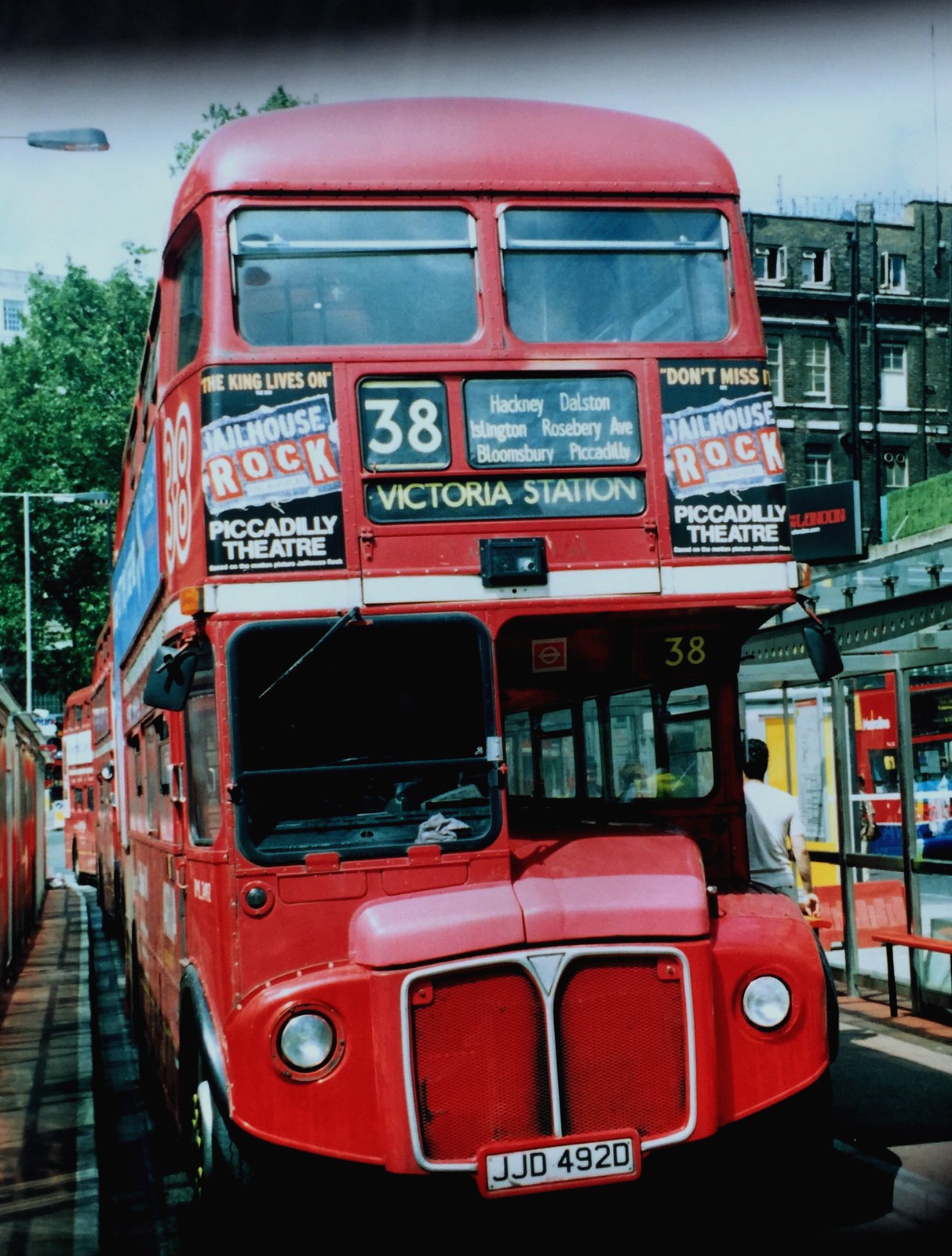The image captures an old-style red double-decker bus prominently positioned in the center, covering the majority of the frame from top to bottom. The bus, with a red and white exterior, features black wheels and has a small squared front bumper. Its front displays a red and silver grill just below a very small windshield area. The destination sign, located on the second level in white on black text, reads "Victoria Station 38," and is flanked by advertisements promoting "Jailhouse Rock" at the Piccadilly Theatre with additional text stating "The King Lives On." The bus's license plate is marked as JJD 492D.

In the background on the right, there's a gray building with balconies and numerous windows, indicating an old structure. Directly below it is a bus stop with a person standing next to red benches. Additional advertisements are plastered on fences adjacent to the bus, which suggest a busy station area. The left side of the background is adorned with green trees and a streetlight, and the sky overhead is relatively blue. Further in the backdrop, other buses are lined up, contributing to the cityscape feel with multiple billboards and varied advertisements enhancing the vibrant urban environment.